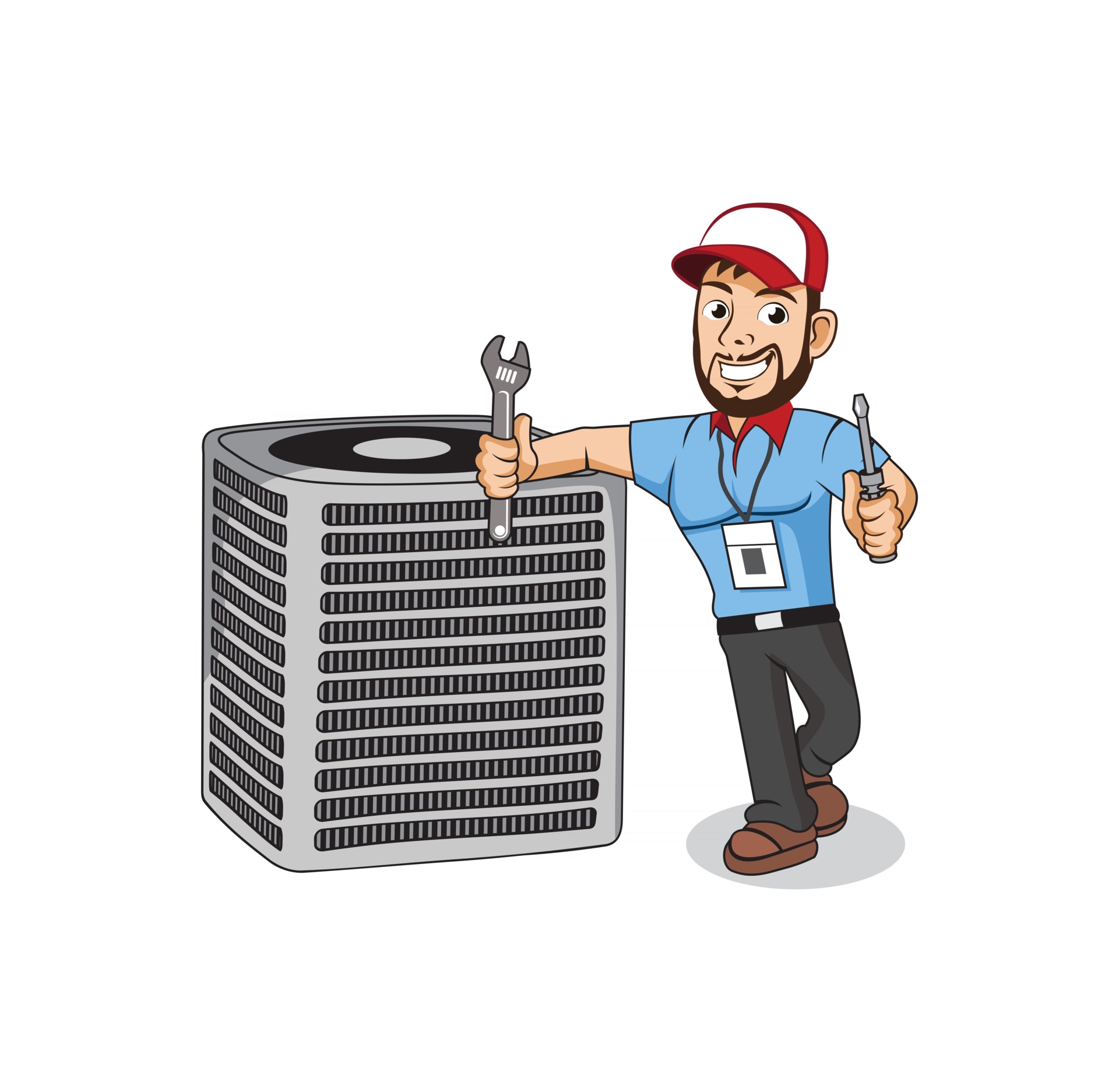The image is a detailed cartoon drawing featuring a Caucasian repairman, likely an AC or radiator technician, standing against a white background. The man is dressed in a uniform that includes a blue short-sleeved t-shirt with a red collar, charcoal-colored pants, a black belt, and brown shoes. He is accessorized with a red and white baseball cap, an ID lanyard hanging around his neck with a white rectangle and a charcoal square in the middle, and has a friendly smile showcasing his white teeth. Additionally, he sports a black beard, mustache, and a bit of black hair peeking from under his cap. In both hands, he holds work tools — a wrench in one and a screwdriver in the other. To his left, there is an outdoor air conditioning unit depicted in various shades of gray and black, nearly cubical in shape with a shadow cast beneath it. This cartoon likely serves as an advertisement and aims to present the repairman as approachable and professional.